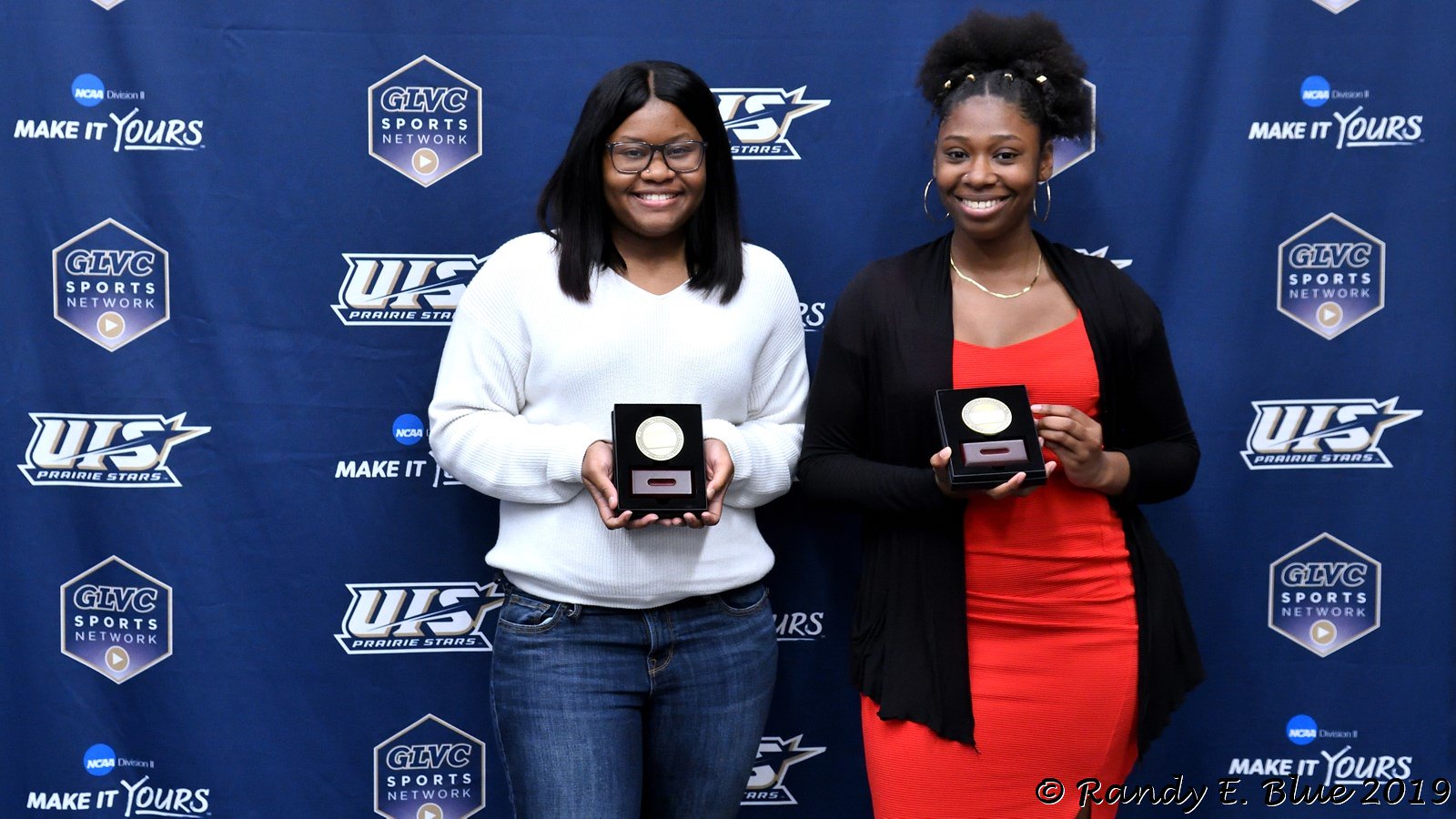In front of a solid blue background patterned with various logos, two African American women stand proudly holding awards, each smiling brightly. On the left, a woman with black-rimmed, square-shaped glasses and shoulder-length black hair parted in the middle wears a long-sleeve v-neck t-shirt with blue jeans. She firmly grasps a thick, rectangular award featuring a silver circle above a gray rectangle. Standing to her right is another radiant woman with her hair styled in a high, puffy ponytail secured with a beaded hair tie. She adorns silver hoop earrings, a headband, a gold necklace, and a red tube dress under a black jacket. She too holds a similar award, positioned carefully in her hands. The backdrop showcases a variety of logos, including "Make It Yours" by the NCAA, GLVC Sports Network, and UIS Prairie Stars, indicating they might be athletes or have some association with these organizations. The scene captures their celebratory moment, radiating joy and achievement.